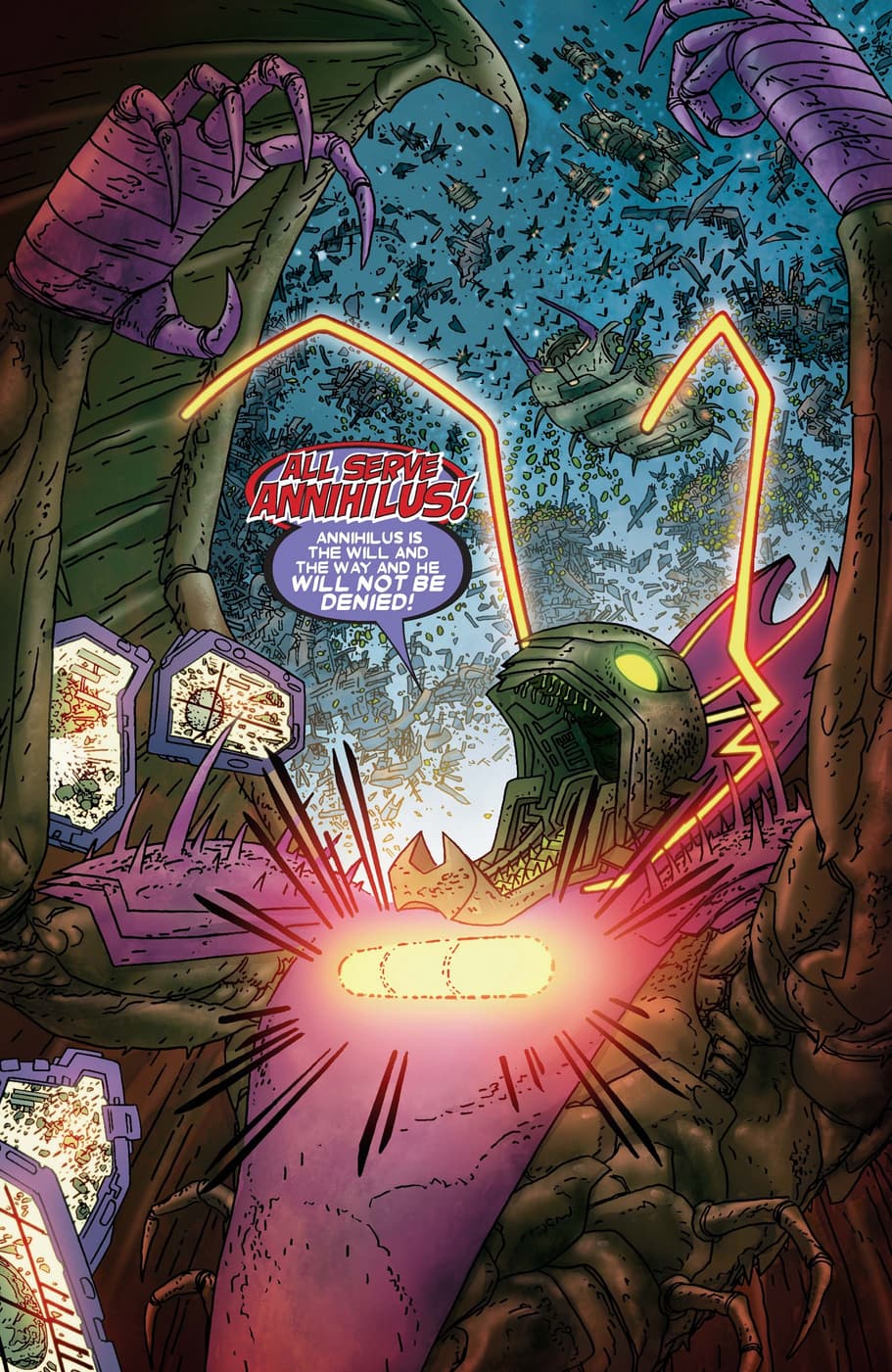The image is a vividly colorful comic book panel set against a deep bluish night sky filled with stars. At the heart of the scene is a monstrous, mechanical insect-like figure, Annihilus, dominating the chaotic space battle. Annihilus, rendered in various shades of green and purple, has anthropomorphic hands with claw-like fingers and glowing yellow antennae arching over his face. His gaping mouth, revealing a tongue resembling a stairway, underscores his menacing presence. His chest glows with a prominent tube-like feature, set within a purple breastplate. The backdrop is alive with numerous ships of different sizes and designs, indicating diverse factions or technologies amidst the conflagration. In the foreground, dramatic text proclaims, "ALL SERVE ANNIHILUS," while a speech bubble emanating from the creature's mouth declares, "ANNIHILUS IS THE WILL AND THE WAY AND HE WILL NOT BE DENIED." The sky is strewn with ships and debris, emphasizing the vast and tumultuous conflict. Monitors or maps with crosshair targets, framed in purple, add to the sense of strategic warfare, as if highlighting Annihilus's control over the ongoing battle from within its chaotic heart.